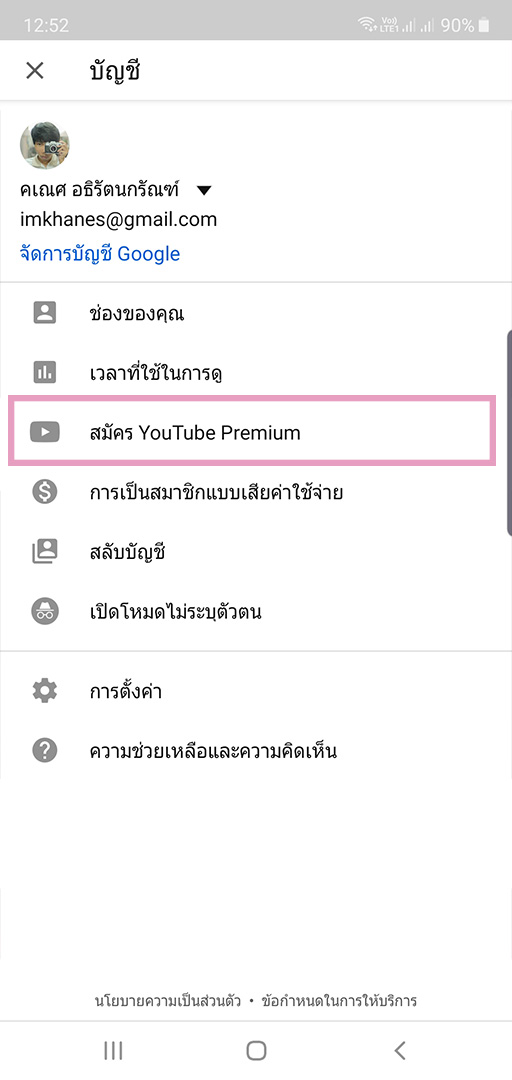In the image, there is a screenshot that appears to be from a digital address book or contact list. The text is predominantly in an Egyptian-style font, giving it a unique aesthetic. At the center of the screen, there is a round profile picture of an individual who seems to be male, characterized by a beard, mustache, and black hair. He is holding a camera in front of his face, which partially obscures his features but leaves one eye visible. Below the profile picture, an email address is listed as imkhames@gmail.com. 

Additionally, the screenshot includes a segment labeled "Google" next to a set of blue characters written in the same Egyptian-style font. A column of various icons, each accompanied by Egyptian characters, is displayed vertically along the screen. One of these icons includes a play symbol and has the English text "YouTube Premium" beside it, indicating a subscription or service related to YouTube. The combination of the unique font and the familiar digital interfaces creates an intriguing and visually engaging composition.